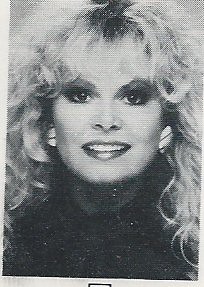This image is a scan of an old black-and-white photograph of Sally Struthers. The photo appears to be a small part of a larger collection, with remnants of writing visible beneath it. It features a close-up of Sally Struthers' face as she looks straightforward with a smile that reveals her upper teeth. She is wearing distinctive round earrings with two horizontal stripes and a dark-colored shirt. Her makeup includes visible lipstick and eyeshadow, complementing her voluminous, wavy, and slightly curly hair, which is reminiscent of the 1980s style. The background of the image is plain white, lacking any discernible details. The photograph itself shows signs of degradation, with visible lines and pixelation, suggesting it is a low-resolution copy, contributing to its rough texture and overall low quality.